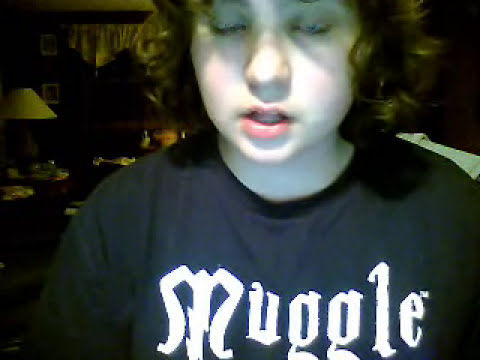This image appears to be a webcam screenshot of a young white girl with shoulder-length, curly dark brown or black hair. She's wearing a black t-shirt with the word "Muggle" written in white, gothic-style letters. She has her eyes closed and her mouth slightly open, giving the impression that she might be in the middle of a conversation. The top part of her forehead is cut off in the image. The background features her living room, which is dimly lit with brown furniture, a white curtain, a white lampshade to the left, and some pictures on the wall. Various items can be seen on a table behind her.